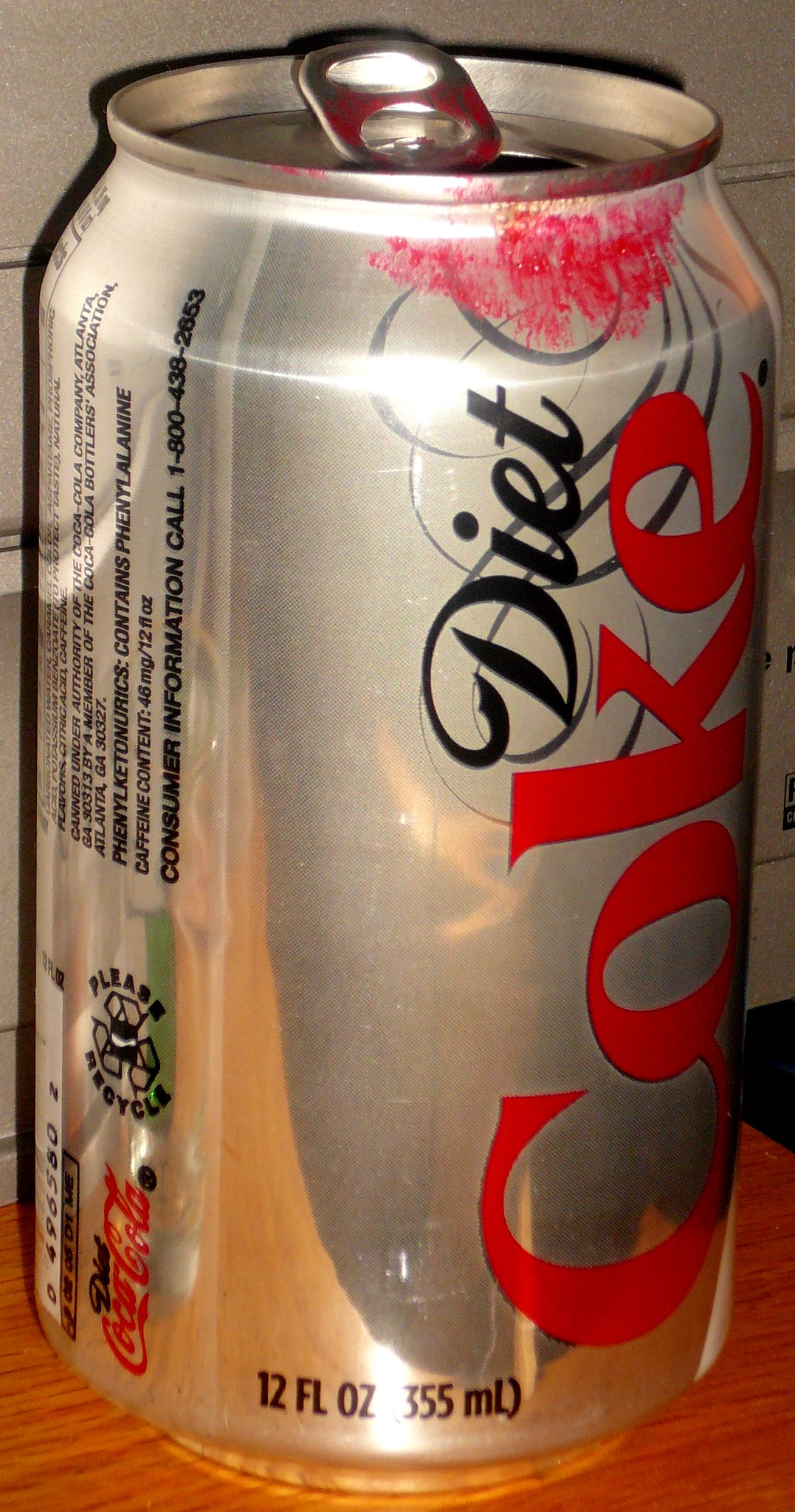A close-up image depicts a standard Diet Coke can sitting on a medium-stained wooden surface. The can, which holds 12 fluid ounces (355 milliliters), is gray with familiar branding details including consumer information and a recycling notice. Light reflections are visible on the can’s surface, and even the photographer's silhouette can be faintly seen. However, the most striking detail is the abundant smears of strawberry red lipstick around the can's rim, particularly concentrated near the opening and the pull tab. This intimate marking suggests the last user had applied the lipstick heavily. The background is somewhat ambiguous, appearing to be a silver-gray or aluminum color, adding to the close-up and focused nature of the shot.